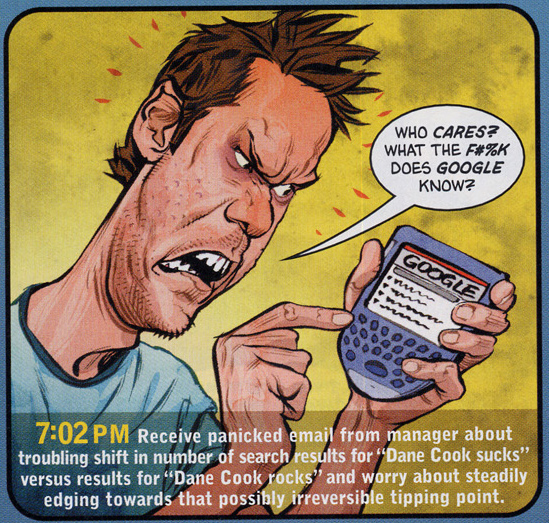The cartoon image depicts a frustrated white man with spiked brown hair on the left-hand side. His face shows anger, and he is dressed in a blue T-shirt. In his hand, he holds a blue device with a large screen, occupying about half of the device, displaying the word "Google." A speech bubble emerges from his mouth, and in black text on a white background, it reads, "Who cares what the F#%K does Google know?" Below this scene, a semi-transparent banner appears, showing the time "7:02 p.m." In white text, the banner reads, "Receive panicked email from manager about troubling shift in number of search results for 'Dane Cook sucks' versus results for 'Dane Cook rocks' and worry about steadily edging towards that possibly irreversible tipping point."